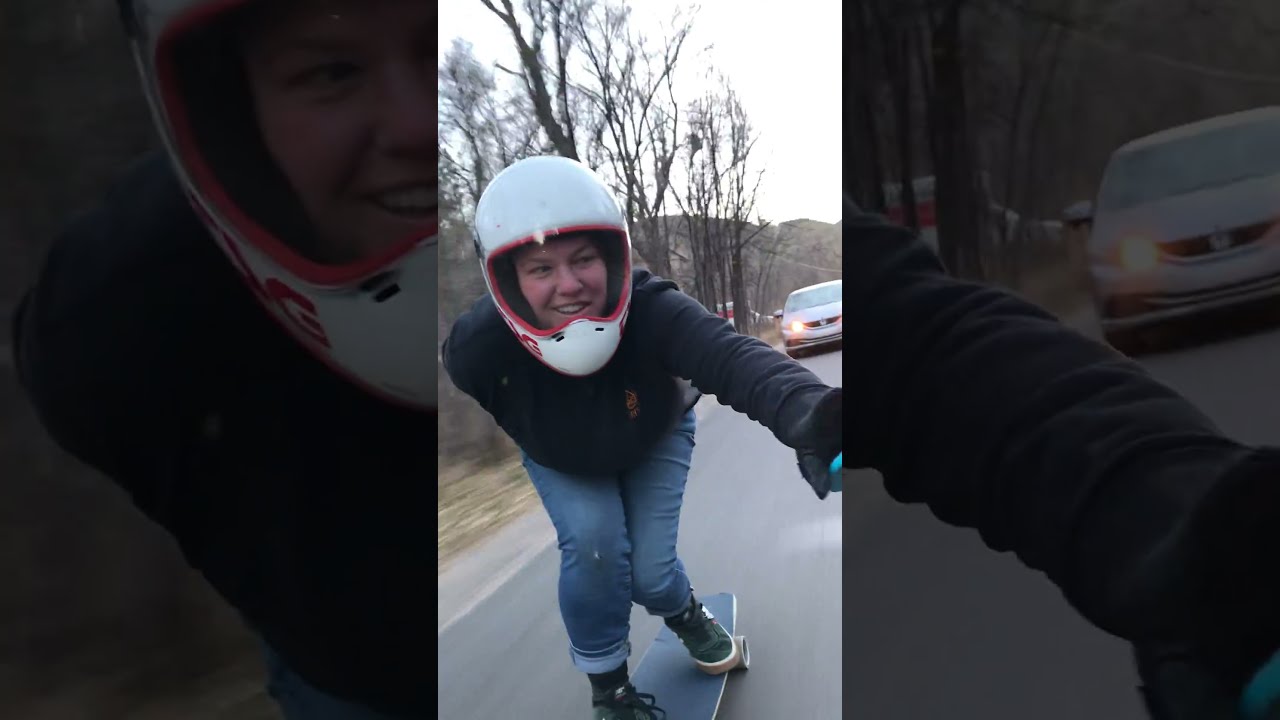This photograph features a woman riding a skateboard on a paved road amidst an outdoor setting. She is positioned in a bent stance, leaning forward with a smile and gazing into the camera. She sports a white full-head helmet with a chin guard, which also has hints of pinkish-orange inside. Her attire includes a black jacket over a blue shirt, blue jeans with rolled cuffs, and black and white tennis shoes. Her hands are tucked behind her back, adding to her engaged demeanor.

The image layout is unique, being taller than it is wide, with solid black borders flanking the left and right sides, creating a vertical strip in the center where the action is captured. On the right side of the image, a part of someone's black and white sleeve is visible, possibly the photographer's, obscuring part of the scene. The background showcases a white sky, brown grass, and some dry trees off to the left side of the road. The wheels of the skateboard are visible as she races downhill, seemingly enjoying her ride in what appears to be a paved trail in a wooded area.